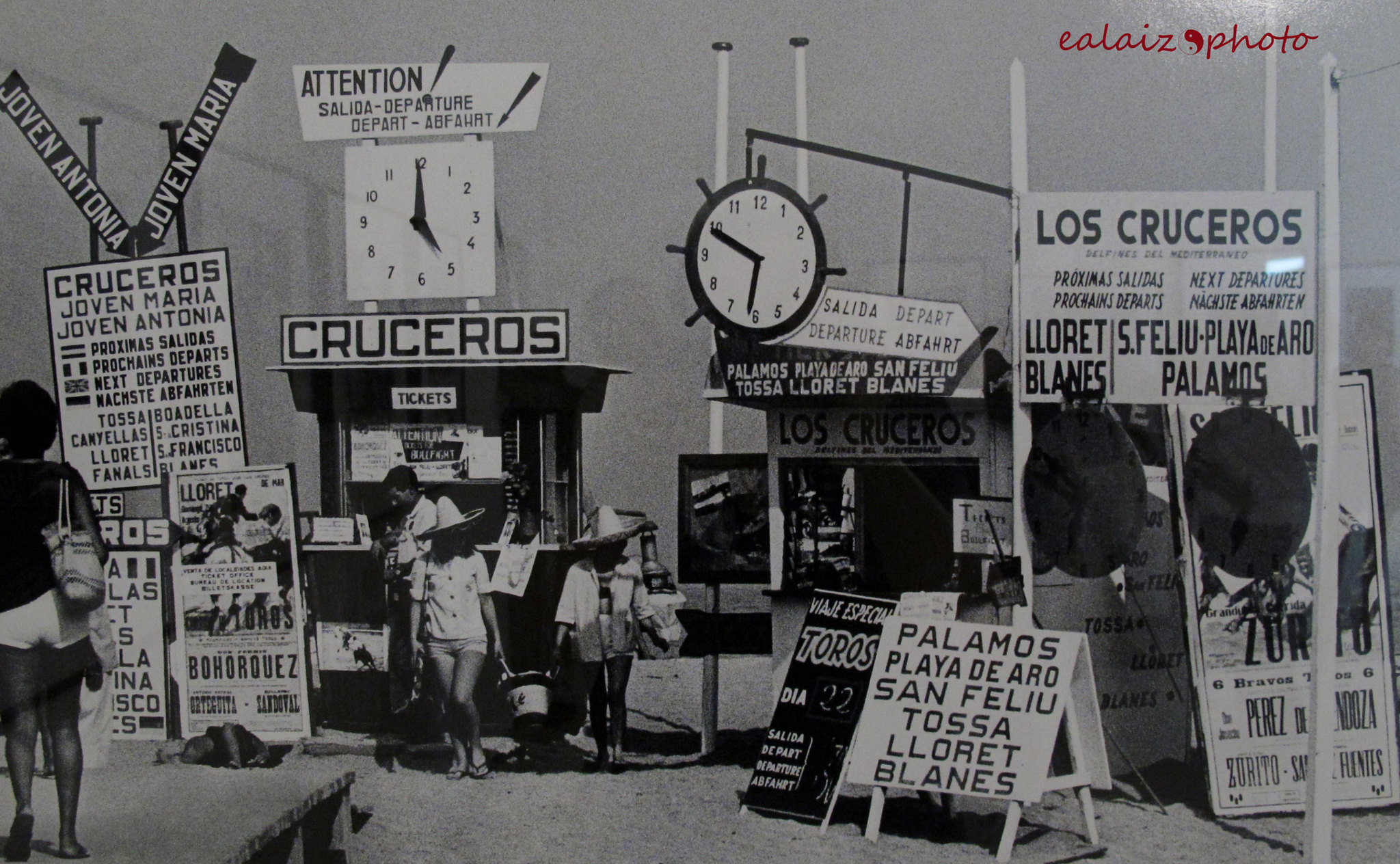In this captivating old black-and-white photograph, a bustling crowd is gathered around various market stands, many of which prominently display the word "Cuceros". The marketplace is alive with activity, featuring a diverse group of people, some wearing hats, engaging with each other and perusing the stands. Notably, there are two large clock towers that stand out amidst the scene, each marking a significant focal point in the photo's composition. Above the lively crowd, a somber, grayish backdrop frames the activity, with an overcast sky adding to the photograph's nostalgic and weighty atmosphere. Scattered throughout the scene are various billboards and signs written in Spanish, affirming the setting to be in a Spanish-speaking country. A red watermark at the top of the image intriguingly declares "A lady's photo", adding an additional layer of mystery and historical context to this evocative snapshot of a bygone era.